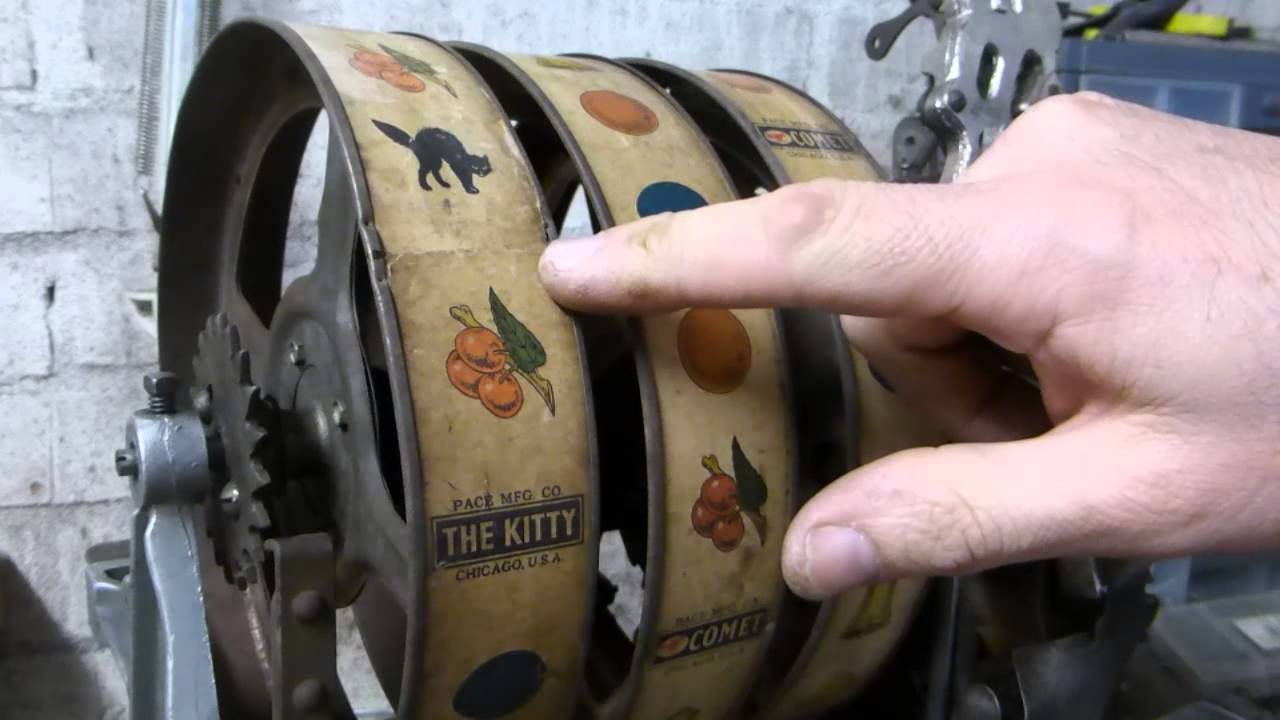This photograph captures a close-up of the inner workings of an antique slot machine, set against a gray stone wall. Prominently featured are three independently rotating metal wheels, each approximately an inch wide, displaying various images such as a black cat, three cherries with a leaf, and three oranges. The images are slightly dirty but still visible. One wheel also features a logo reading "Pace MFG Co.," along with "KITTY" in all caps and "Chicago USA" beneath it. From the right side of the image, a white-skinned hand extends, pointing specifically at the orange picture on the leftmost wheel. The wheels are attached to metal rods that suggest they are part of a larger gear mechanism typical of old slot machines.